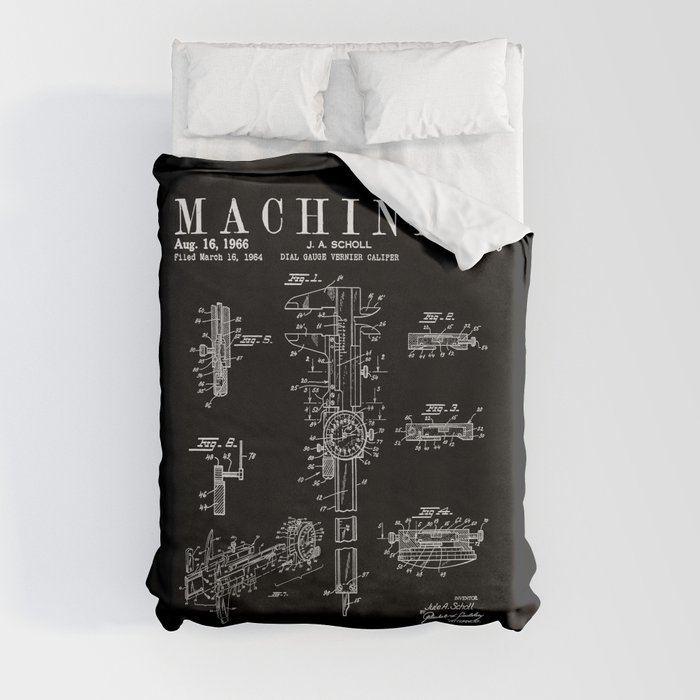This detailed image captures a bed, centrally positioned, adorned with a black duvet cover marked with intricate blueprint designs. The bed, likely queen or king-sized, features two white pillows at the head, suggesting a sense of symmetry and comfort. The white main sheet contrasts with the black duvet, which is slightly folded at the top right corner, revealing a glimpse of the underlying layer. The blueprint design on the duvet illustrates various mechanical parts, though the exact nature of the machine is indeterminate. The visible text "MACHI" hints at the word "MACHINE," flanked by the dates August 16, 1966, and March 5, 1964. The name J.A. Scholl appears prominently, indicating a possible association with the depicted design. The background is grey, and additional machines, rendered in the same white outline style, flank the central mechanism, enhancing the technical theme of the image.